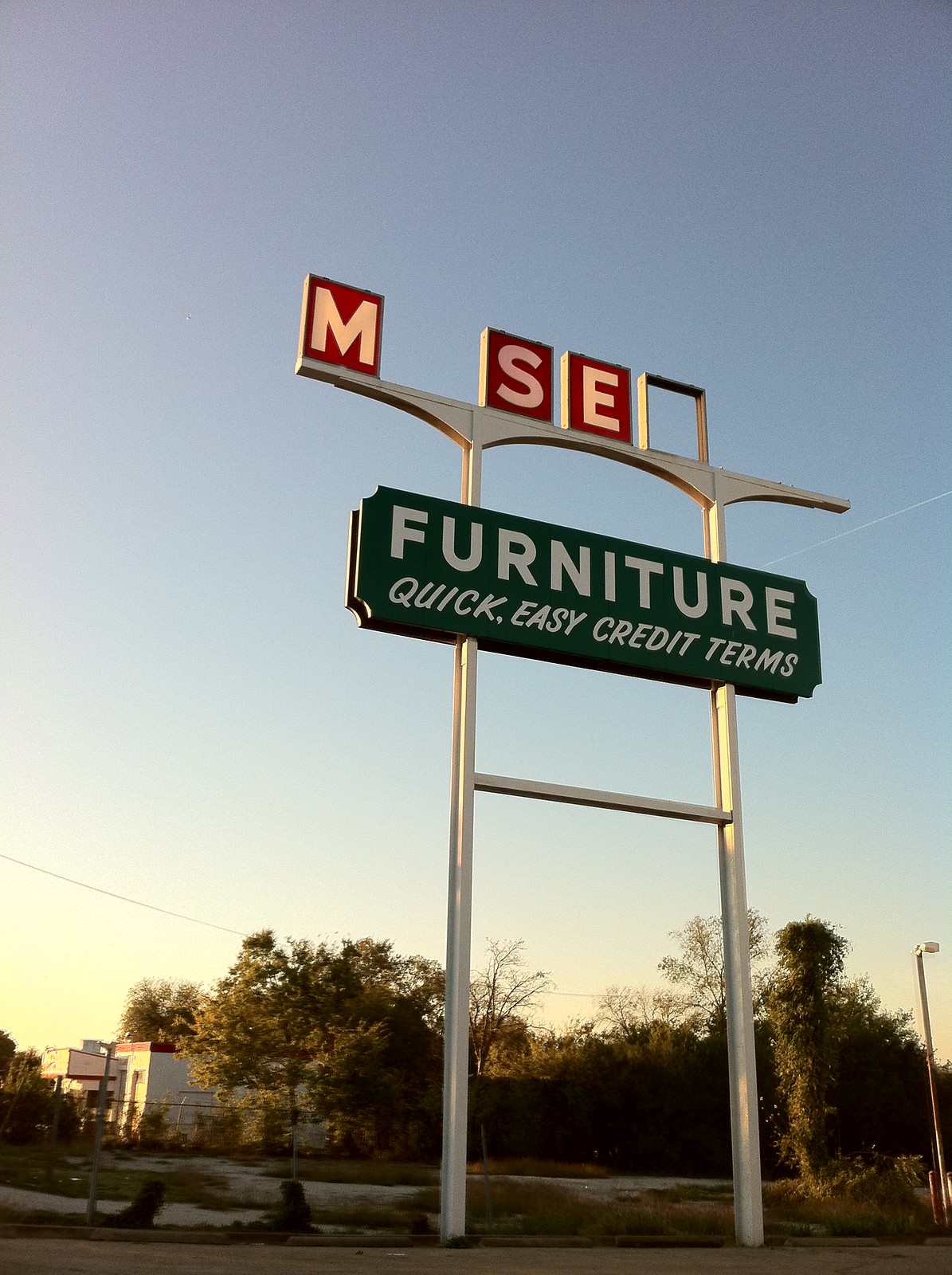The photograph captures a tall, retro-style roadside sign, likely from a furniture store, against a clear blue sky. The sign, standing around 10 to 12 feet tall, is supported by silver metal poles forming an H shape, and is situated on a green grassy area with various buildings, possibly houses, visible in the background. The top section of the sign features large white letters "M", "S", and "E" on a red background, with missing letters indicated by blank spaces. Immediately below, a rectangular sign with curved notches on its corners displays the words "FURNITURE" followed by "QUICK, EASY CREDIT TERMS" in white text. The overall design includes both silver and gray elements, with the structure resembling a combination of a football post and a decorative bridge-like shape, contributing to its retro appearance.